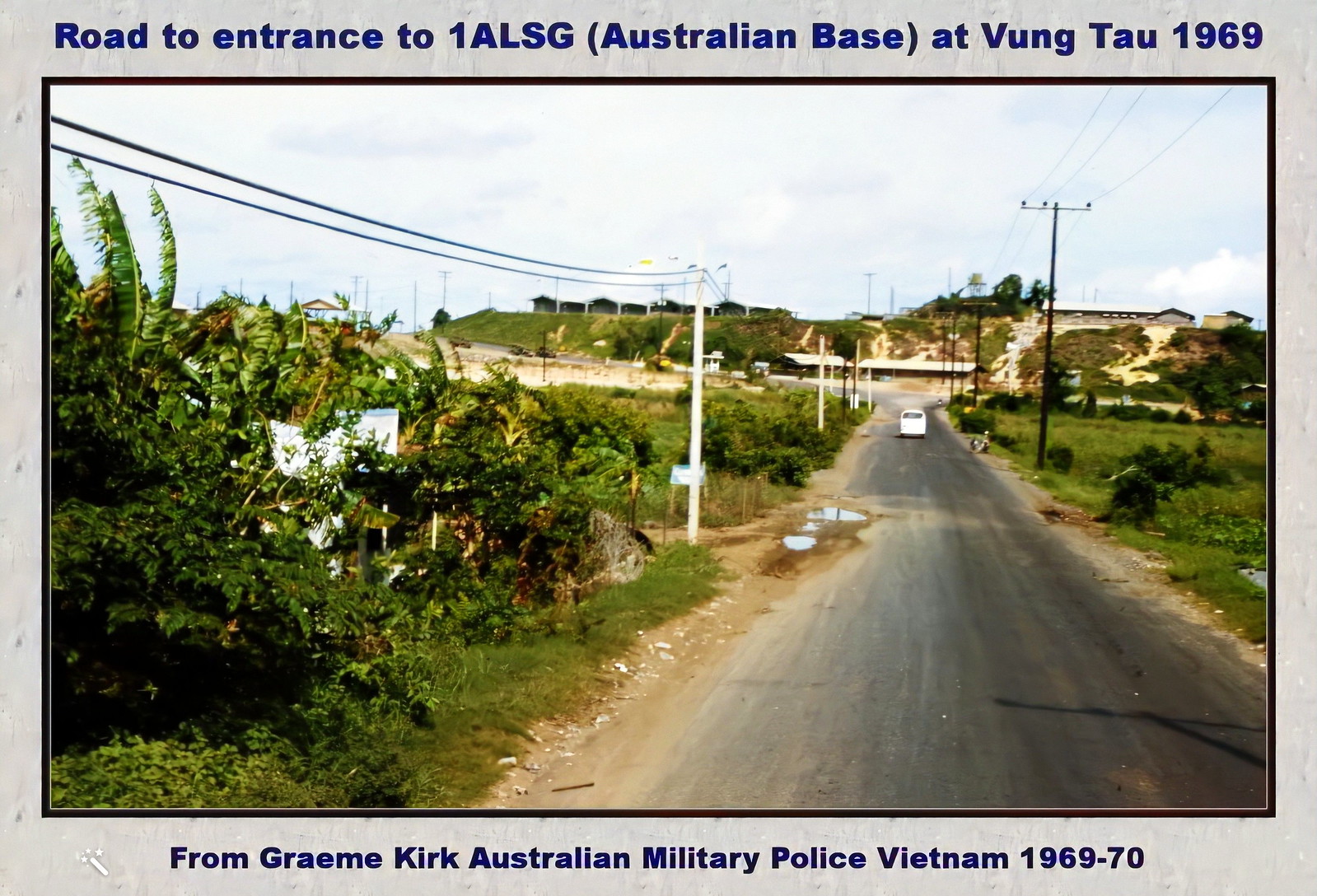The image is a historical photograph of the road leading to the entrance of 1 ALSG, an Australian base at Vung Tau in 1969. It includes a digital border with blue text at the top reading, "Road to Entrance to 1 ALSG (Australian Base) at Vung Tau, 1969," and at the bottom, "From Graham Kirk, Australian Military Police, Vietnam, 1969-70." The border has a whitish, marbled texture, highlighted by dark gray lines framing the photograph.

The road itself, paved in asphalt with dirt edges, curves left and is flanked by telephone poles and wires. The left side of the image features dense vegetation and flora, while the right side is grassy with smaller bushes. In the background, small buildings—possibly houses or tented overhangs—and a hillside are visible, with the road skirting around the hill rather than ascending it. The photograph also shows a white van, which appears to be moving away from the camera.